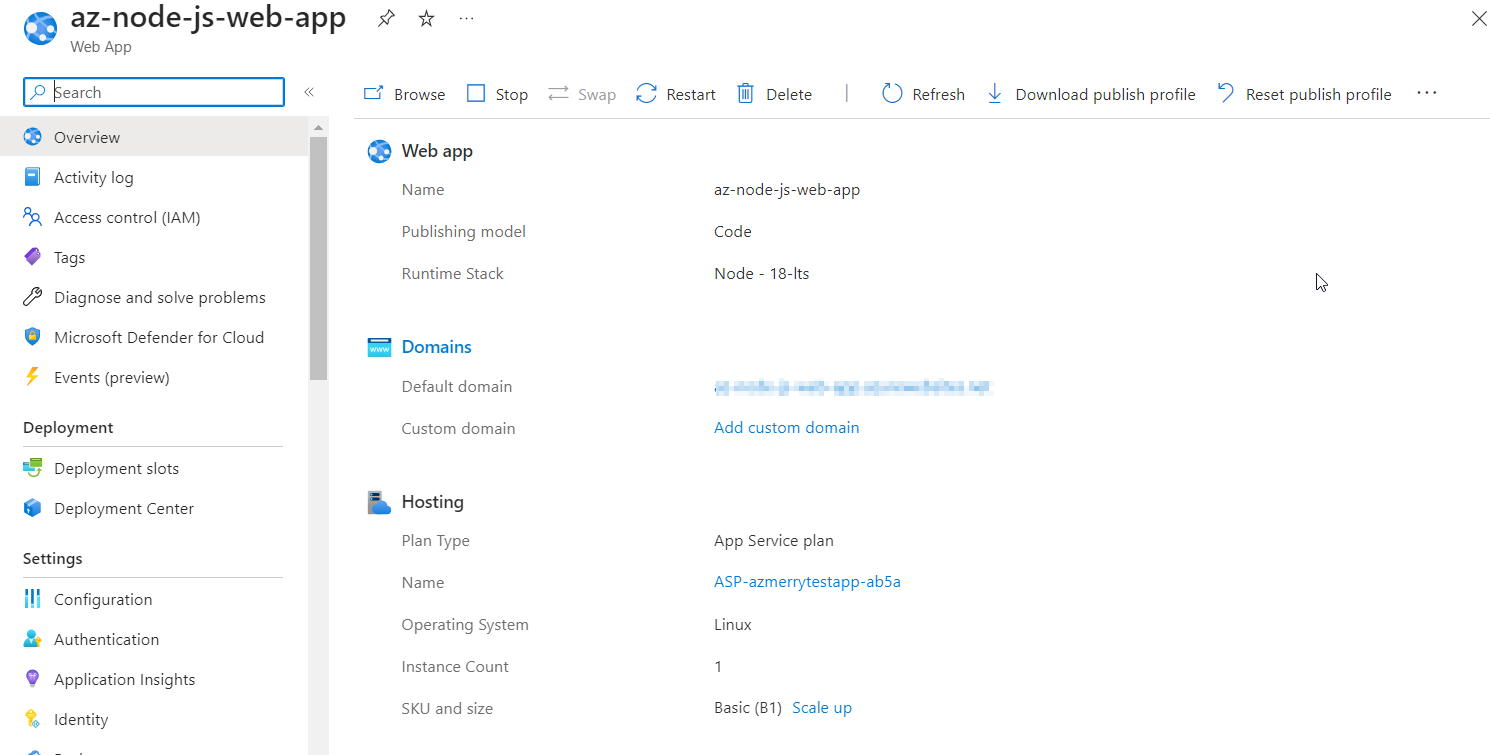A detailed screenshot of a website showcasing the management interface for a Node.js web application named "az-nodee-js-web-app." At the top, the application’s name is prominently displayed in bold. Below that, there is a search bar under the label "Web App."

Running vertically on the left side of the interface is a navigation pane featuring various management options represented by both text and icons. The first section is "Overview," followed by "Activity Log." Next is "Access Control (IAM)," succeeded by "Tags." There is a wrench icon that leads to "Diagnose and Solve Problems," and a shield icon for "Microsoft Defender for Cloud." A lightning bolt icon indicates the "Events, Preview" section. Further down, there are sections for "Deployment," including subsections "Deployment Slots" and "Deployment Center," both marked in black. "Settings" follows, under which are four visible tabs: "Configuration," "Authentication," "Application Insights," and "Identity." The fifth tab is partially cut off but clearly indicated.

On the right side of the interface, there is a broader section labeled "Web App," where users can input details such as Name, Publishing Model, and Runtime Stack. Below, there are sections for "Domains," categorized into "Default Domain" and "Custom Domain." At the bottom of this section, a "Hosting" category is also visible. The clean and organized layout ensures users have easy access to various functionalities for managing their Node.js web application effectively.